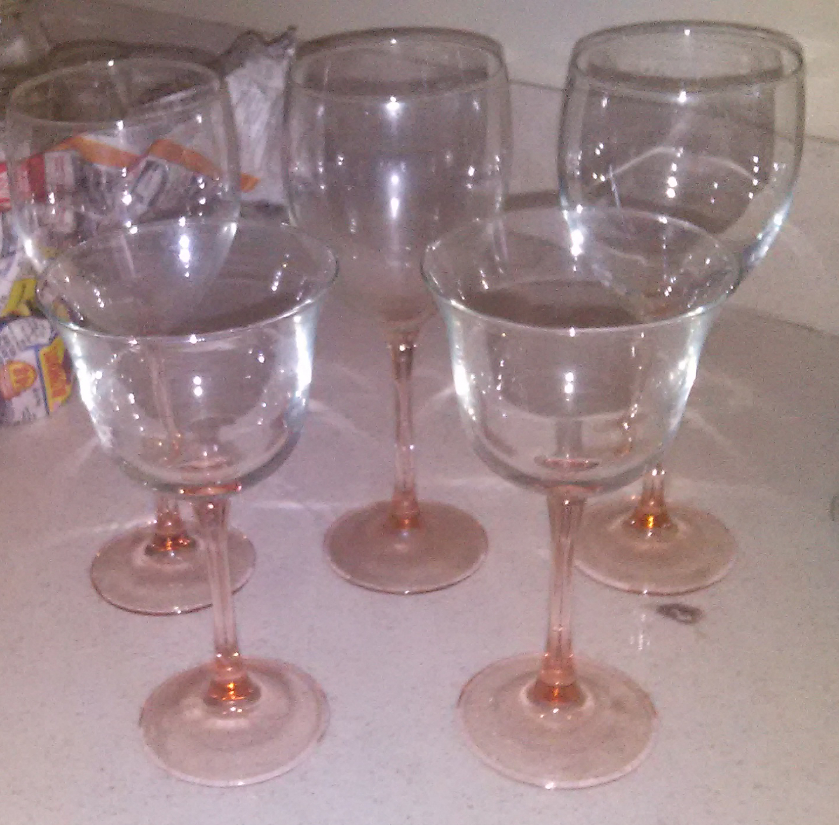A color photograph captures five crystal-clear wine glasses positioned on kitchen worktops, which are glazed with a pinkish hue. The wine glasses, all with matching tall stems, feature a distinctive pinky-salmon color. The arrangement includes three standard wine-shaped glasses placed at the back and two glasses at the front, which are reminiscent of goblets with their rolled edges and wider mouths. These two front glasses could even double as elegant candle holders. Behind the back glasses, a crumpled newspaper is faintly visible, adding a casual touch to the scene. The worktops also have a noticeable black spot, suggesting it might have been burnt at some point. The background consists of a white wall, emphasizing the clean and detailed arrangement of the glasses.